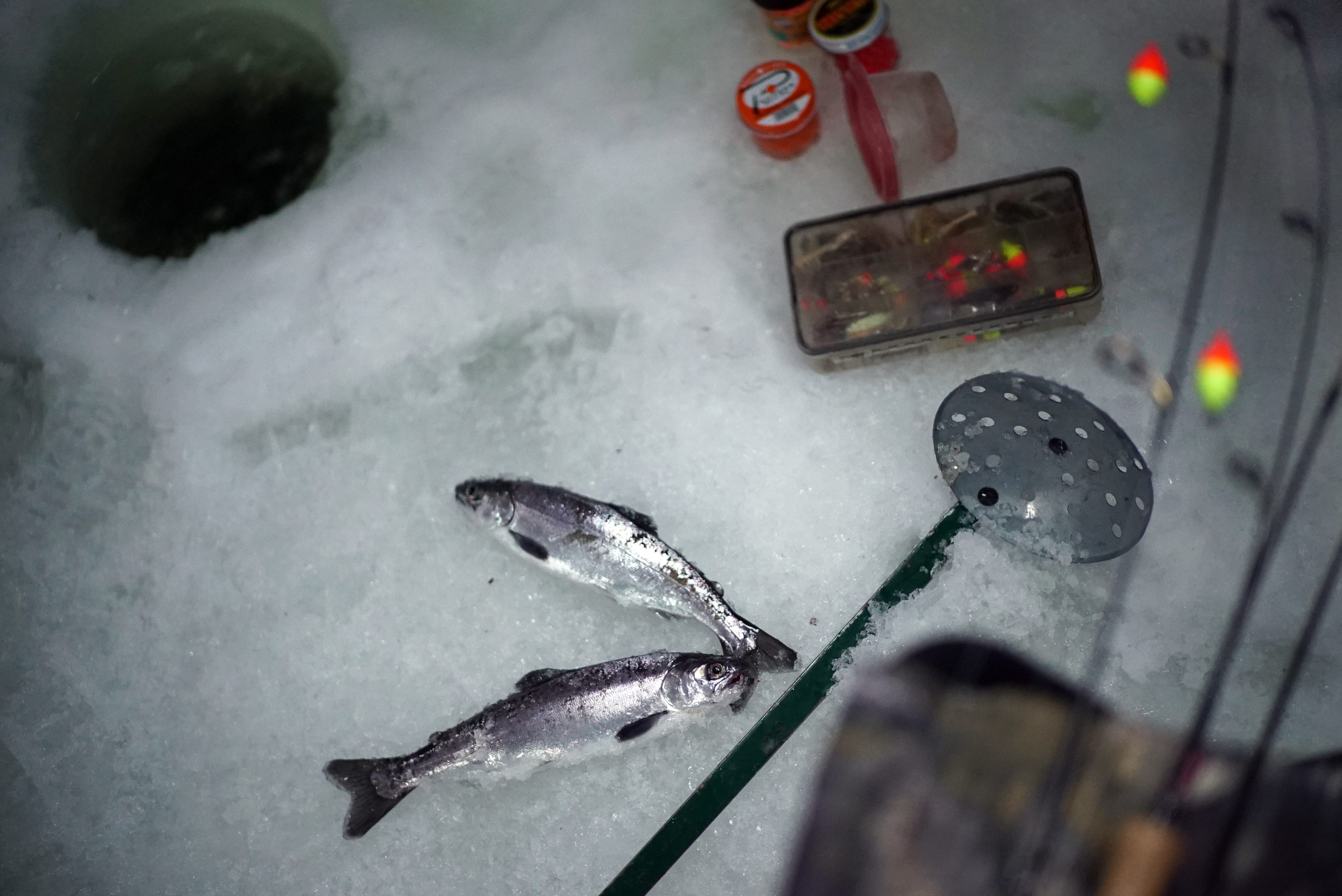The image captures a small, ice fishing scene on what appears to be a snowy, icy surface, likely on a lake or river during winter. In the center, there's a noticeable fishing hole surrounded by various fishing gear. Prominently, there are two silver-colored fish, possibly sockeye salmon, resting near an array of tools. Among the tools, there's a red and silver metal ladle with perforated holes at the bottom, used possibly for scooping ice. Nearby, a see-through tackle box reveals various small fishing tools and hooks. Above the tackle box, there are three small cylindrical containers: two with red bodies and black tops, and one with an orange body featuring white text. To the right, an empty cylindrical container with a red cap is visible. The scene is slightly blurred on the right side with flashes of neon and orange hues. The predominant colors in the image include shades of silver, white, red, neon, orange, brown, and black, indicating a cold, wintry environment. Adding to the scene's authenticity, a fishing line can be seen alongside the tools, reinforcing the ice fishing theme.